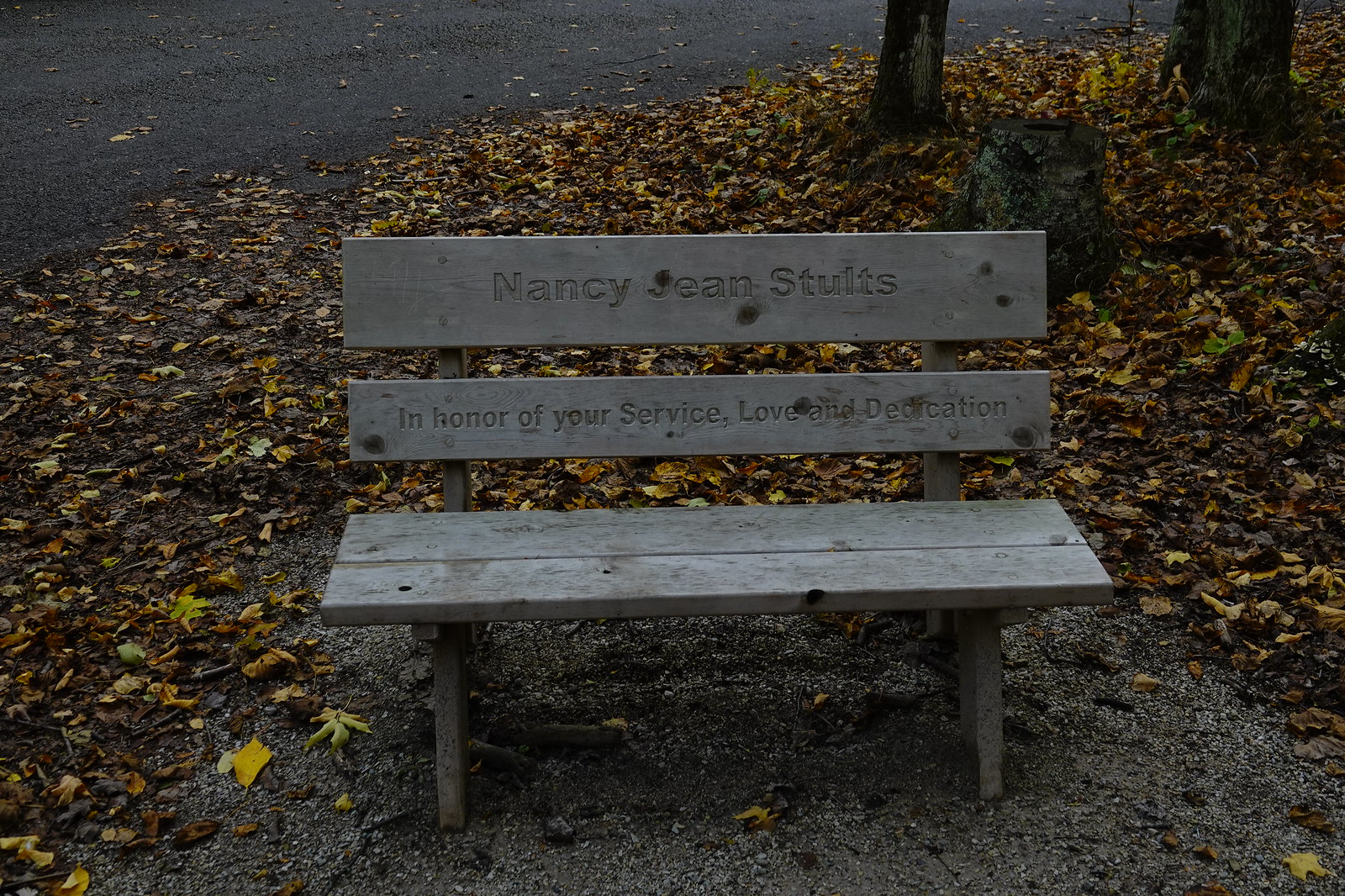This is a photograph of a wooden bench in an outdoor setting, possibly a park. The bench has a light grey, almost whitish color and features an engraving on the back support that reads: "Nancy Jean Stoltz, in honor of your service, love, and dedication." The bench is placed on a ground that is covered with a mix of green sand and dry leaves in shades of yellow, brown and green. Behind the bench, there are a few tree trunks and rocks visible, suggesting a natural, somewhat wooded area. The bench is positioned next to a black pavement or road, and the photo appears to have been taken during late evening or at night, as it is quite dark. The overall scene is serene and unoccupied, emphasizing the quiet tribute inscribed on the bench.